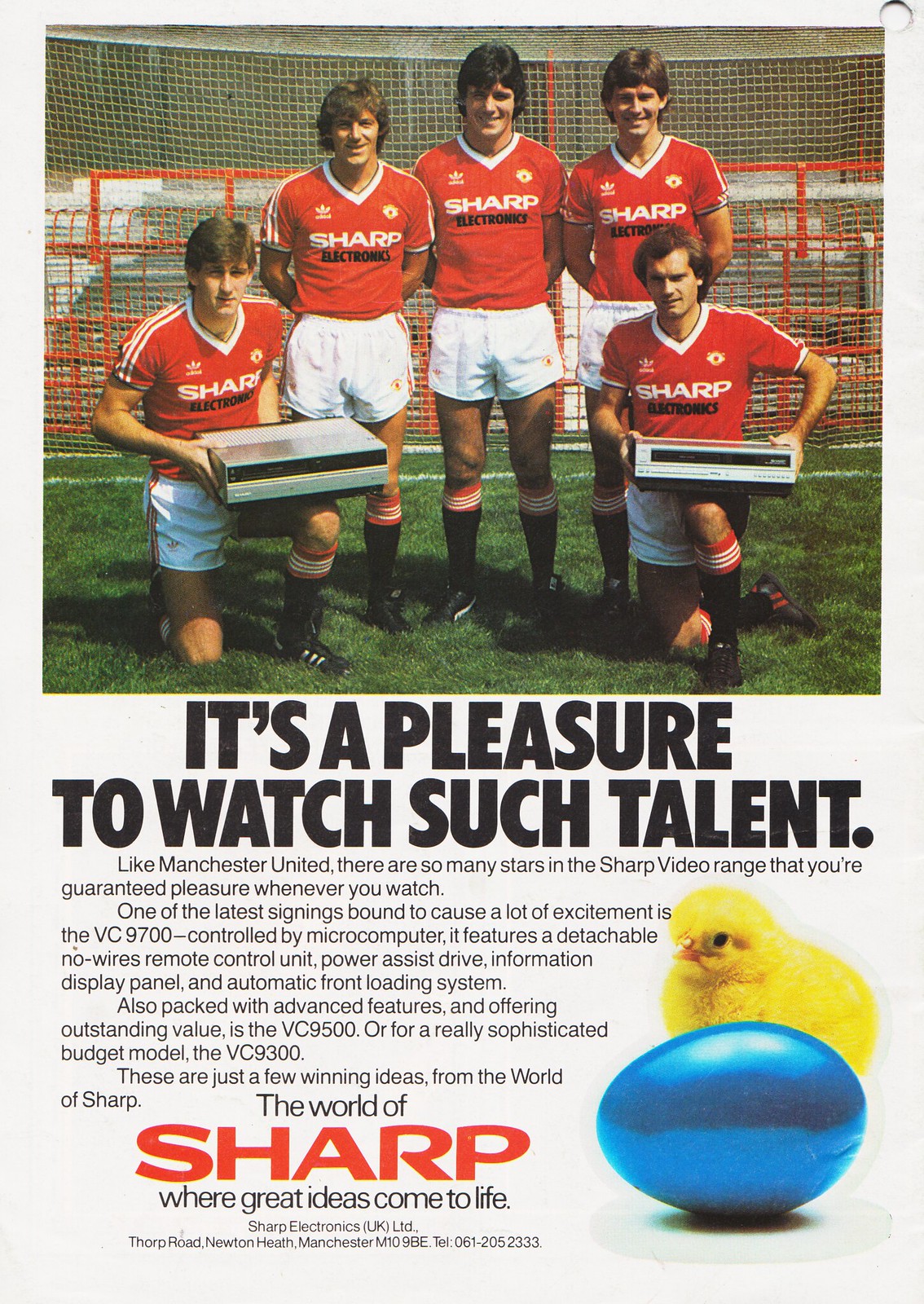This image is an advertisement from an older magazine, featuring a promotional scene for Sharp Electronics. The top half shows five soccer players, dressed in matching red shirts that read "Sharp" in white lettering and "Electronics" in black, paired with white shorts. Three men stand in the back while two kneel on either side in the front, each holding a large silver box resembling an old-school VCR, highlighting the vintage nature of the ad. The players are positioned on a grassy field with a soccer goal in the background. Above them, bold text declares, "It's a pleasure to watch such talent."

Beneath the players, the advertisement contains detailed text, likening the array of Sharp's video products to the many stars of Manchester United, ensuring customers a pleasurable viewing experience. It spotlights several models: the VC9700, featuring microcomputer control, a detachable, wireless remote, power-assist drive, information display panel, and automatic front-loading system; the feature-packed and value-offering VC9500; and the sophisticated budget-friendly VC9300.

In the lower right corner of the ad, a small, eye-catching image shows a yellow chick standing in front of a blue egg, accompanied by the tagline, "The world of Sharp, where great ideas come to life."